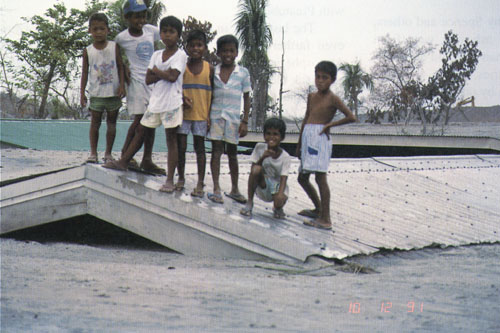In this evocative photograph taken on October 12, 1991, in a tropical South American community, seven young children stand atop a silver metal roof amidst severe flooding. The water level has risen almost to the top of the roof, with less than a foot of space remaining. The children, aged around five or six, are lined up at the roof's edge, smiling and looking towards the camera. They wear old, casual clothing, predominantly white shirts and shorts, with one child in a yellow tank top adorned with a blue stripe and another child on the right standing shirtless in white shorts. None of the children are wearing shoes. Surrounding them, other rooftops, including a green roof to the left and another metal roof to the back right, poke through the floodwaters. In the distance, the landscape is dotted with tropical trees, possibly including palm trees, against a backdrop of lush greenery. The poignancy of the scene is heightened by the children's precarious perch and the floodwaters enveloping their environment.